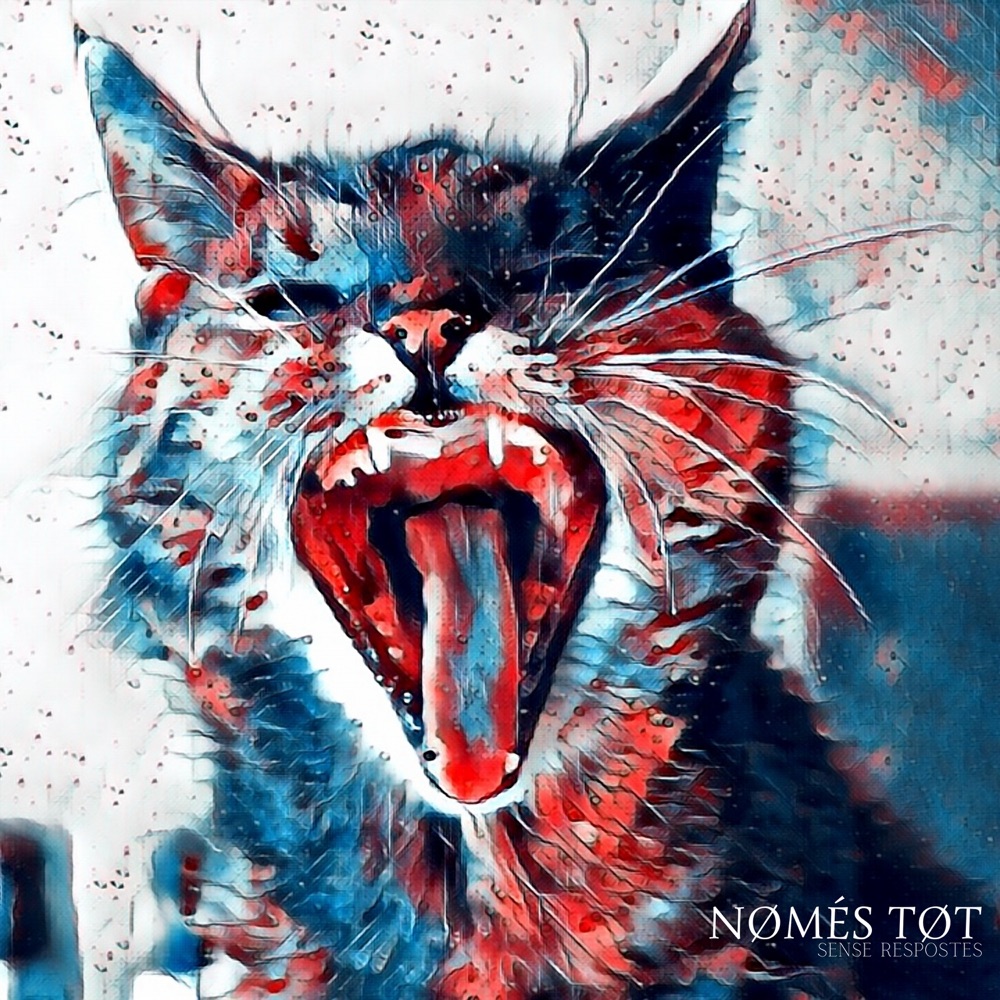This is an artistic depiction of a yawning cat, rendered in a vibrant palette of red, white, and blue hues. The cat's mouth is wide open, showcasing sharp upper teeth and a tongue that is predominantly red with streaks of blue. Its fur is a mix of red, blue, and black, with a particularly dark-toned ear on the left side of the drawing. The cat's eyes are solid black, and it has long, prominent white whiskers. The background consists of a white canvas scattered with small red and blue specks, creating a dynamic, splash-like effect. The bottom right corner of the image features some text, which appears to read "Nomestot, Sense Reposits," though the exact wording is unclear. The artwork stands out with its patriotic color scheme and detailed portrayal of the cat in a unique and expressive style.